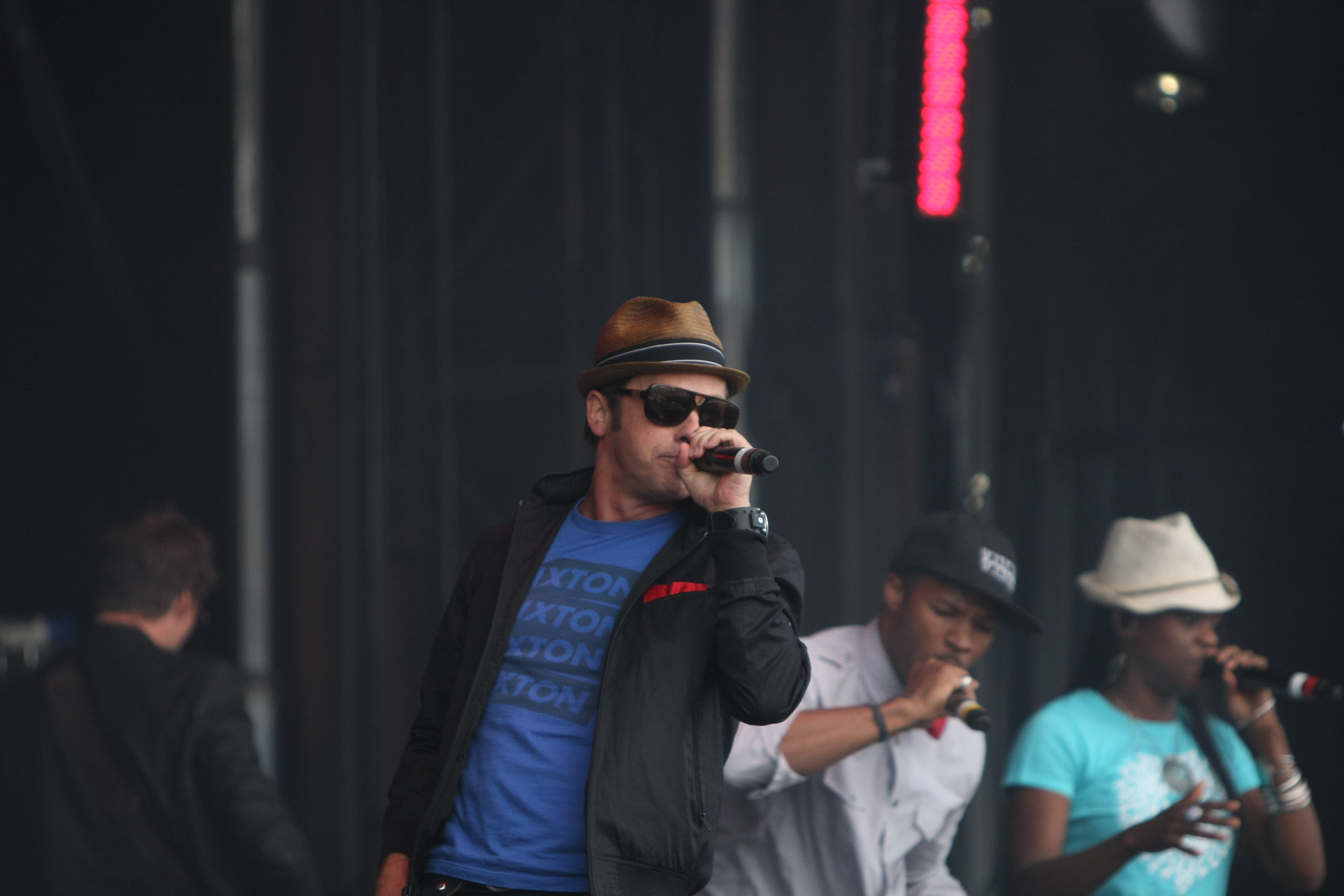In this photograph, a quartet of performers is captured mid-performance on a dimly lit stage with a black backdrop. The central figure, a white male, is prominently featured in the foreground, holding a black microphone to his face. He wears black sunglasses, a brown hat with a white and black stripe around the rim, a blue t-shirt partially obscured by a black jacket with a red handkerchief peeking out from the pocket. Standing slightly behind him to the right is a black male with a black baseball cap adorned with white words. He too holds a microphone close to his mouth, wearing a gray button-down shirt that seems to be complemented by a red bow tie. Next to him, a black female singer dons a white fedora and turquoise t-shirt with a white pattern. Her ensemble is accessorized with a gray necklace and multiple gray bangle bracelets on her left arm. She also holds a microphone, singing into it. At the far left, slightly in the background, appears the back of another white male with dark hair in a black suit jacket. The stage lights cast a reddish-pink hue, adding a dynamic element to the otherwise dark setting, which includes a hanging vertical light in the top-right corner.